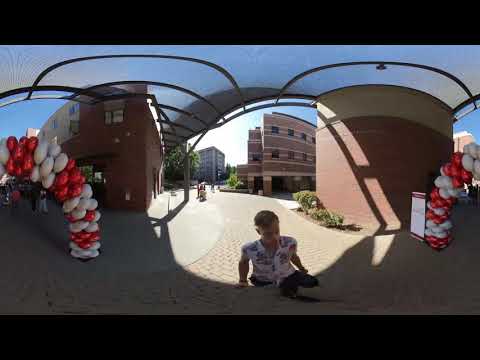A detailed photograph captures a sunny day in a city courtyard, featuring a man with side-parted hair walking on a terracotta brick walkway. The man is positioned centrally under two large balloon arches in an upside-down horseshoe shape, featuring red and white balloons on either side of him. The scene is bathed in bright sunlight, casting significant shadows due to the clear, blue sky. Surrounding the courtyard are three- to four-story tan and red brick office buildings. The ground is interspersed with patches of greenery and shrubbery. Additional background details include other people in the area, such as a person pushing a baby in a stroller, suggesting a communal or event-like atmosphere possibly suitable for a farmer's market or job fair. The man appears to be approaching or entering a tent-like area that permits some sunlight through, contributing to the numerous shadows cast in the photo.